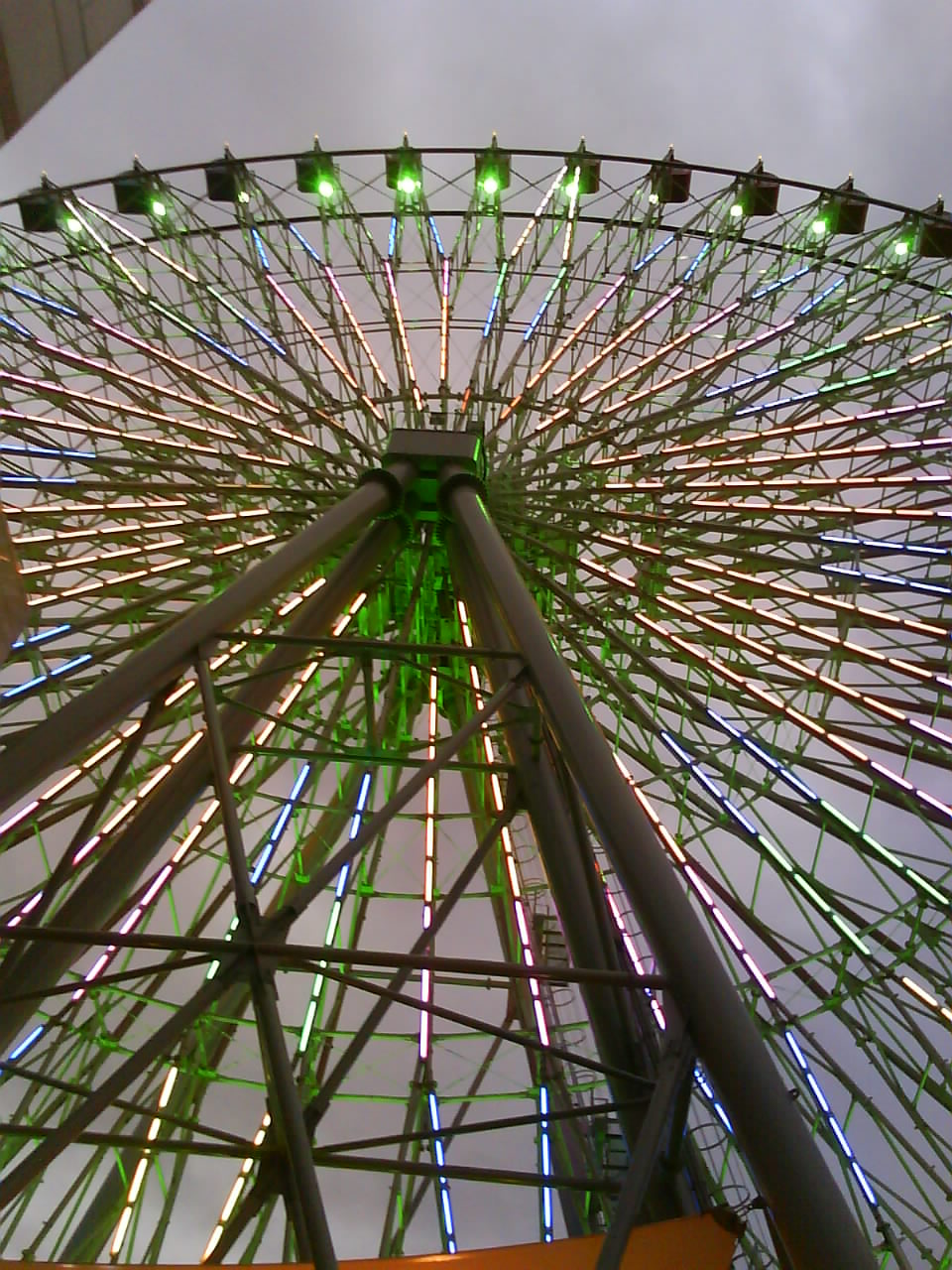This photograph captures a striking upward view of a towering Ferris wheel, dominantly occupying the frame against a backdrop of blue sky. The Ferris wheel is supported by four dark gray steel legs that converge towards its middle, creating a robust structural base. The wheel itself is adorned with numerous green lights, which illuminate the entire structure, including each of the orange-colored Ferris wheel cars. These green lights highlight the intricate framework, casting a vibrant glow that enhances the visual appeal. The perspective from below emphasizes the grandeur and height of the Ferris wheel, with its base looming large in the foreground and extending skyward. All around, the bright green lights and the dark metallic elements create a captivating contrast, making the Ferris wheel the focal point against the serene sky.